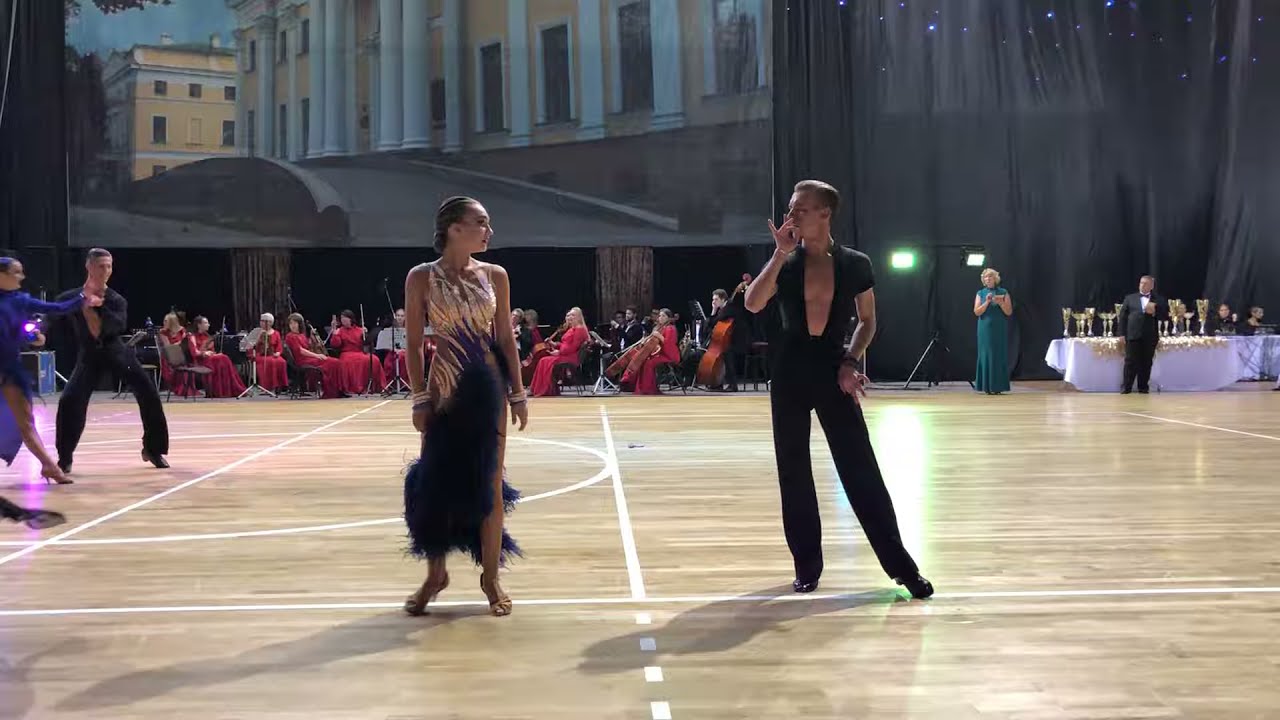In an indoor gymnasium with light brown wood flooring and white sectioning lines, the primary focus is a dance couple poised mid-dance at the midline. The left dancer, a woman with dark brown hair pulled back into an ornate bun, wears a gold sequined sleeveless dress that cuts high on her left hip, transitioning to a black, feathered bottom. Golden bangles adorn her wrists as she looks at her male partner to her right. He has light-colored, slicked-back hair and wears a tight-fitting, black short-sleeved shirt with an open front revealing his chest, paired with long black pants. His right hand is posed in front of his face, with his fingers forming a circle.

To the left, another dancing couple mirrors similar attire. The woman sports a purple long dress, and her partner wears the same black outfit as the primary male dancer. In the background, from the left to just past the midline, an orchestra clad in red for the women and black for the men occupies the space, their string instruments evident. To the right, a long table covered with a white tablecloth displays trophies, attended by a man in a black suit and tie, and a woman with blonde hair donning a long green gown. Behind them, black curtains frame a projected image of buildings, setting the stage for what appears to be a dance competition.